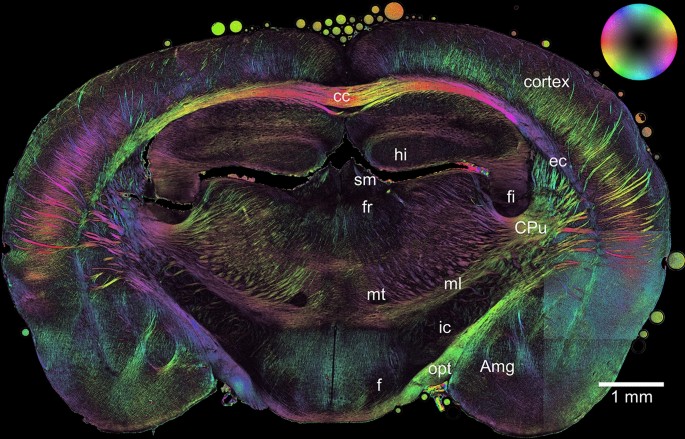The image appears to be a detailed and colorful brain scan displayed on a black background. It shows a sagittal view of a human brain, sliced to reveal the inner structures but viewed from a side profile perspective. The brain scan is brightly colored with iridescent hues ranging from yellows and reds to purples and greens, highlighting various regions. Numerous parts of the brain are labeled in white text, including abbreviations such as cortex, CC, HI, SM, FR, FI, EC, CP, OPT, and AMG, among others, predominantly on the right side. A color wheel representing the rainbow spectrum is located in the upper right corner, while a scale indicating a measurement of 1 millimeter is positioned in the bottom right corner. The image presents a vivid, almost artistic representation of brain structures, making the intricate labeling and coloration both scientifically informative and visually striking.